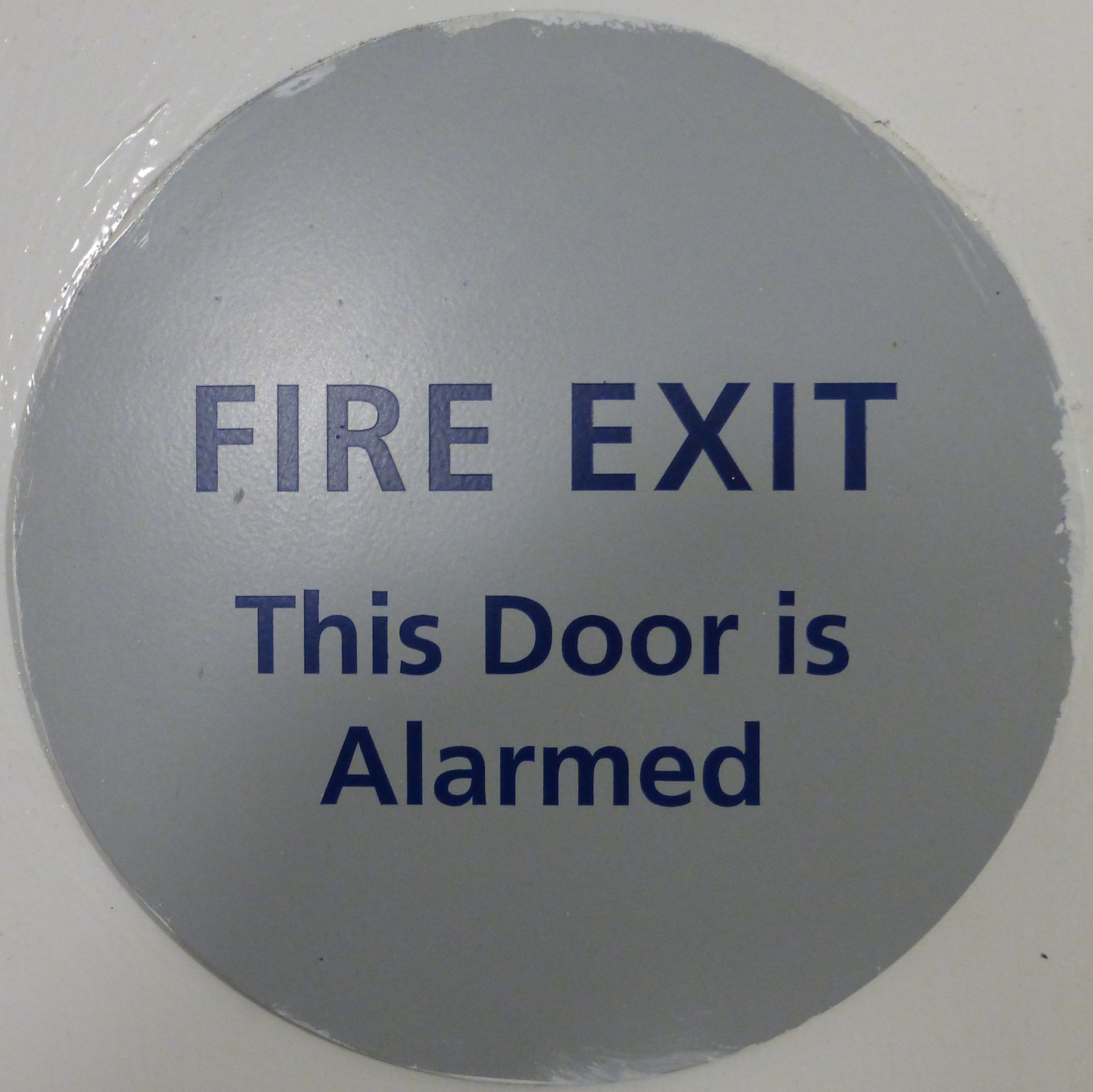The image depicts an alert sign featuring a dominant dark gray circle against a light gray background. Centered within the circle are large, navy blue, capital letters that read "FIRE EXIT," with smaller text below that states "THIS DOOR IS ALARMED." The entire sign appears to be mounted on or painted on a surface that has a glossy white finish, though the gray circle itself and the text within it possess a more matte appearance. The edges of the gray circle look slightly streaky or blurred, as if the lighter gray paint around it was sloppily applied or is peeling off to reveal the darker gray beneath. There is also a small black speck visible near the bottom right corner of the image, which could be dirt or another imperfection on the surface.